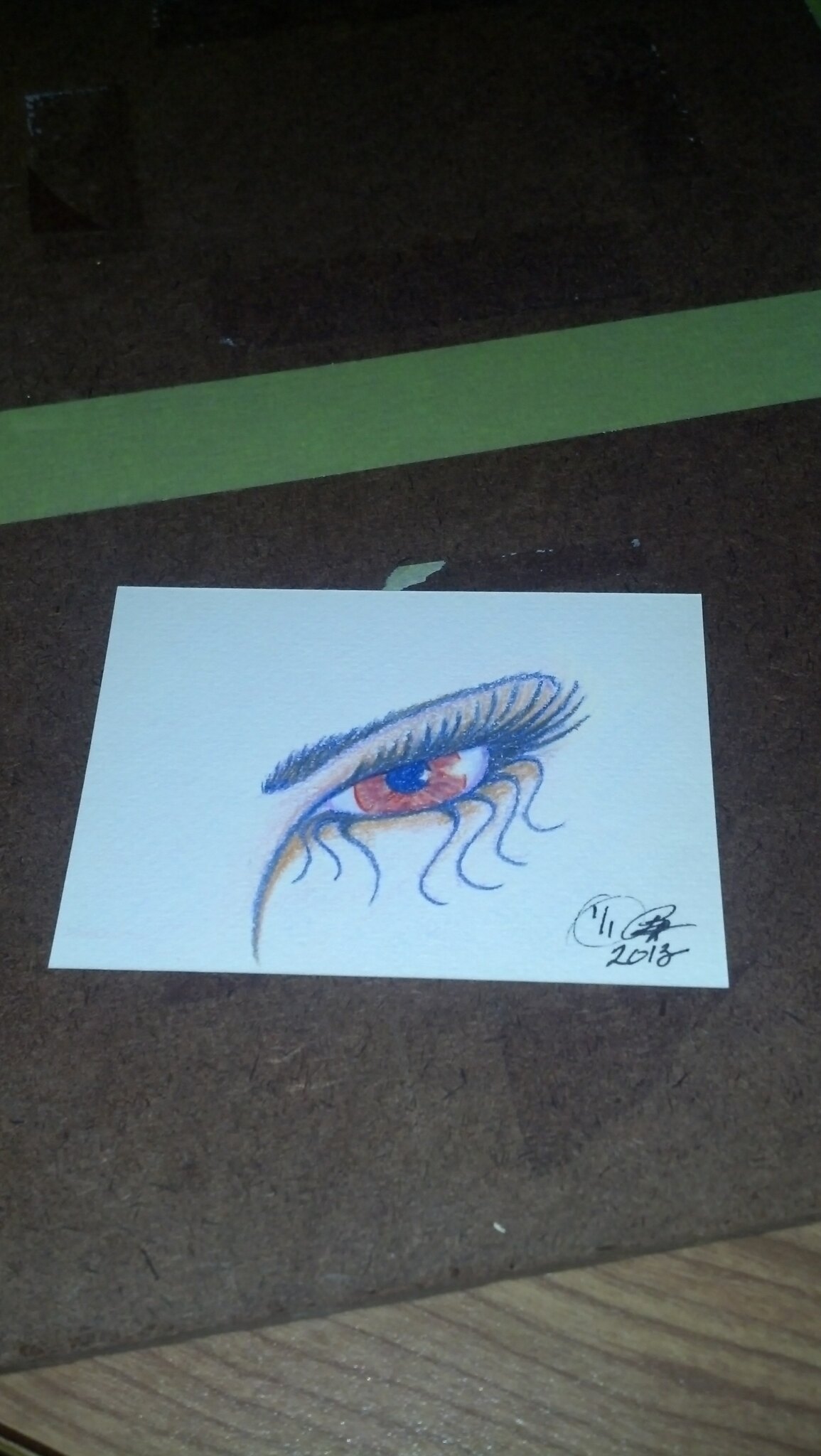This is a colored pencil drawing centered on a woman's eye, showcasing a sultry and interested look. The iris is a captivating blend of orange, brownish, and reddish hues, with a hint of hazel, while the pupil reflects a small glint of light. The eye is framed by long, meticulously drawn eyelashes—seven curly ones on the bottom that stand out—and a carefully brushed eyebrow with some shading between them. The drawing is sketched on a plain white, horizontal sheet of computer paper. An unreadable signature and the date "1-1-2013" are inscribed on the bottom right. The background comprises brown wooden floors, and the paper rests on a brown object with a green stripe at the top.